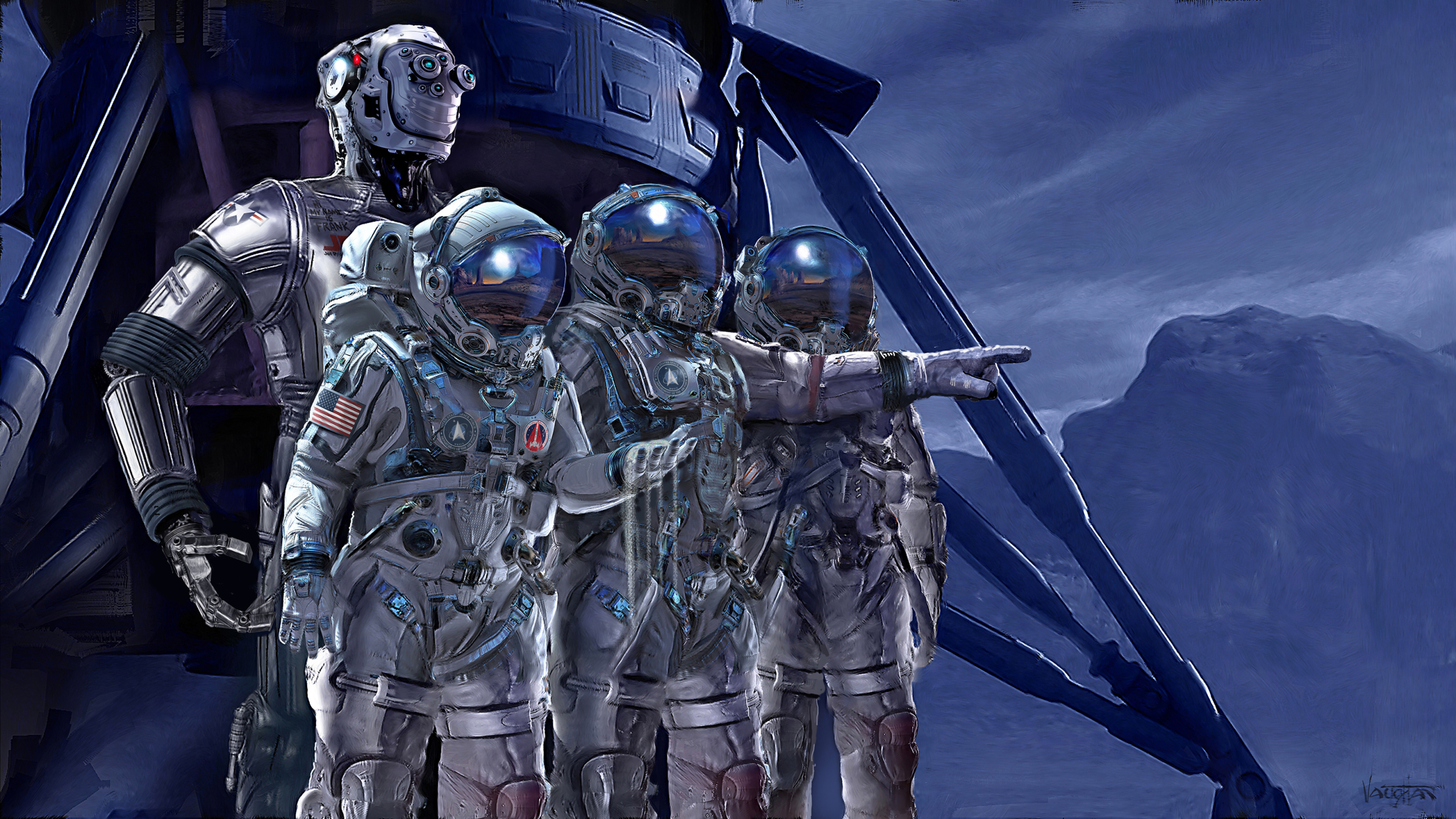In this detailed colored pencil or graphic drawing, shaped in a rectangular format roughly six inches wide and three inches high, the scene is set on an alien planet. The background is dominated by shades of blue, creating a hazy, atmospheric sky with distant mountains barely visible through the mist. 

On the left side of the image stands a futuristic, metallic spacecraft designed like a tripod with three protruding legs, suggesting a recent landing. Propped sturdily on the ground, this space-aged vehicle adds to the theme of exploration.

In front of the spacecraft, three astronauts in light gray uniforms with visors down are aligned closely side by side. The central astronaut points towards the right, drawing the attention of the others, including a robust robot standing behind them. This chrome-plated robot, identified as "Frank," towers over the astronauts by at least a head. Frank features distinctive eyes on its forehead and detailed metallic hands and fingers.

Accentuating the scene, one astronaut on the left appears to be examining the ground, with sand or dirt flowing through their hand, and sports an American flag on their suit. The overall color palette, dominated by blues and grays, lends a cohesive, otherworldly ambiance to this moment of interstellar discovery and collaboration.